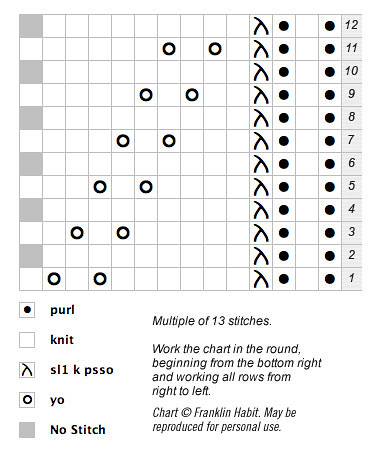The image is a detailed knitting pattern chart, designed on a checkered grid with a white background and some gray boxes. The grid is organized centrally within the image, measuring 14 by 10 squares. Along the farthest right column are numbers descending from 12 to 1. Adjacent columns feature a variety of symbols: solid black circles, empty squares, and an angled T shape rotated 45 degrees, among others. These symbols are used to indicate different knitting instructions. Below this chart, there is a key explaining the symbols: a solid black dot signifies purl, an empty square signifies knit, an angled T signifies S-L-1-K-P-S-S-O, an open circle indicates YO, and a solid gray square means no stitch. Text at the bottom provides additional instructions, stating that the pattern should be worked in the round beginning from the bottom right and proceeding left to right across rows. This chart is meticulously designed for knitters to follow and is illustrated clearly with black text and symbols for easy reading.